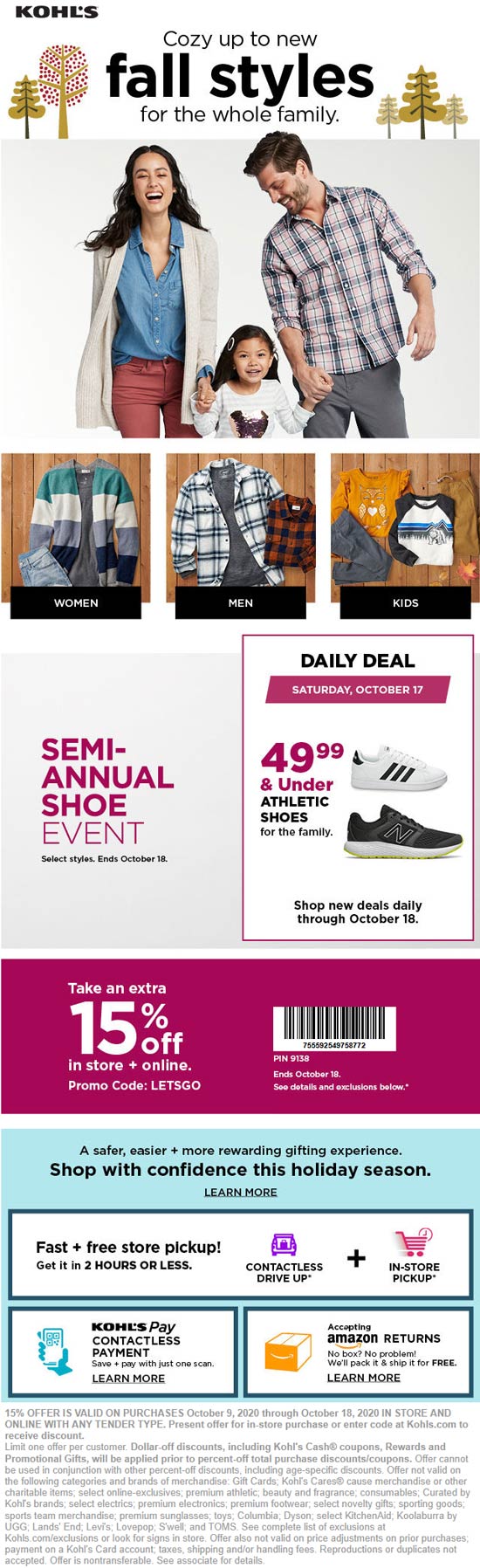**Screenshot of Kohl's Advertisement**

The advertisement, set against a clean white background, prominently features the name "Kohl's" in capital black letters at the top left. Directly below the logo are two animated, hand-drawn trees, contributing to an autumnal theme. To the right of the trees, the ad encourages viewers to "Cozy Up to New Fall Styles," with the phrase "fall styles" highlighted in larger black letters. Below this message, it states, "For the whole family."

To the right, three more animated trees continue the fall aesthetic. Beneath these illustrations, a photograph displays a cheerful trio: a young man, a young woman, and a small child, all holding hands and smiling. The man, who has short brown hair and is White, wears a checkered button-down shirt with gray pants. The woman, with long brown hair and an appearance suggesting Asian heritage, is dressed in a cardigan sweater over a blue work shirt and pink pants. The child, also with long brown hair and a barrette, mirrors the Asian appearance and wears a white shirt adorned with a pink heart.

Under this image, there are three distinct sections featuring clothes arranged on a wooden background. The sections are labeled "Women," "Men," and "Kids."

- The "Women" section displays a cardigan, a gray shirt, and blue jeans.
- The "Men" section showcases a checkered shirt over a gray t-shirt and a red and black checkered shirt.
- The "Kids" section includes a pair of gray pants, a dark yellow shirt with hearts, and a white shirt with a bear design and dark blue shoulder accents. Additionally, a tan piece of clothing is included.

Below these sections, there is a promotion for shoes, headlined by "Daily Deal Saturday October 17th $49.99," highlighting athletic shoes for the family. To the left, the ad mentions the "Semi-Annual Shoe Event" with a long pink bar announcing "Take an Extra 15% Off," accompanied by a barcode.

At the bottom, a blue section reassures customers to "Shop with Confidence this Holiday Season," mentioning benefits such as rewards, free store pickup, contactless drive-up, Kohl's Pay, contactless payment options, and acceptance of Amazon returns.

The very bottom of the ad contains several store policy notes and legal disclaimers, including statements like "Limit one offer per customer" and "See complete list of exclusions."